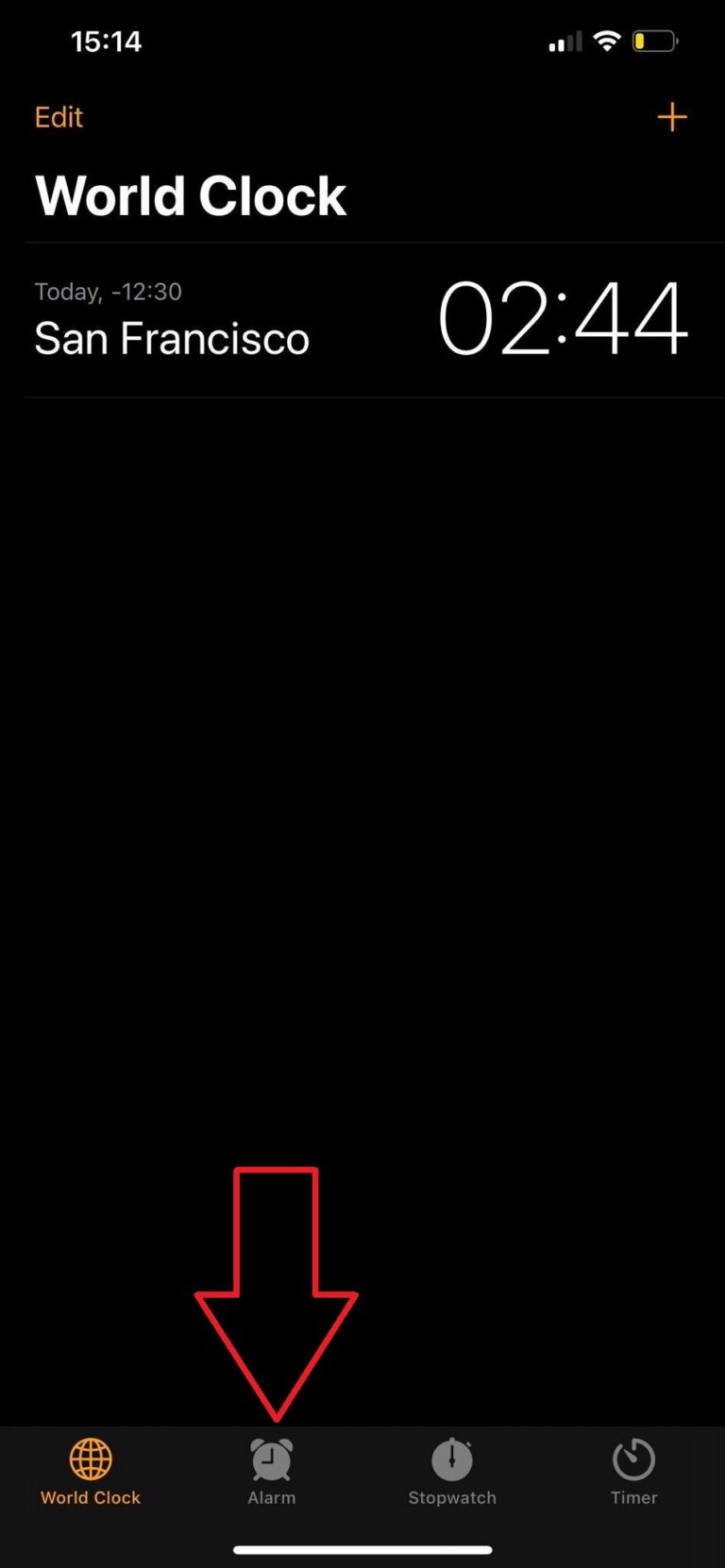The image, viewed on a mobile device, appears to be a screenshot from the alarm setting interface on a smartphone. The background is a deep, jet black, providing a stark contrast to the other elements on the screen. The lower portion of the screen features a dark gray bar with a set of four icons: "World Clock" is highlighted in orange and marked by a globe icon, while "Alarm," "Stopwatch," and "Timer" are displayed in gray.

A prominent, photoshopped red arrow is pointing toward the "Alarm" icon, drawing attention to it. 

In the upper left corner, the time is displayed as "15:14." Adjacent to the time, icons indicate the device's status: a "two out of four" data connection, a "three-bar" Wi-Fi signal, and an almost depleted yellow battery bar.

Just below these indicators, in orange text, the options "Edit" and a "+" sign are situated on the far left and right respectively.

A white section labeled "World Clock" follows underneath, showing the current time in San Francisco as "02:44."

Finally, at the very bottom edge of the screen, there is a white bar intended for sliding to minimize the interface. The overall composition of the image suggests a purposeful focus on the alarm setting feature of the smartphone.